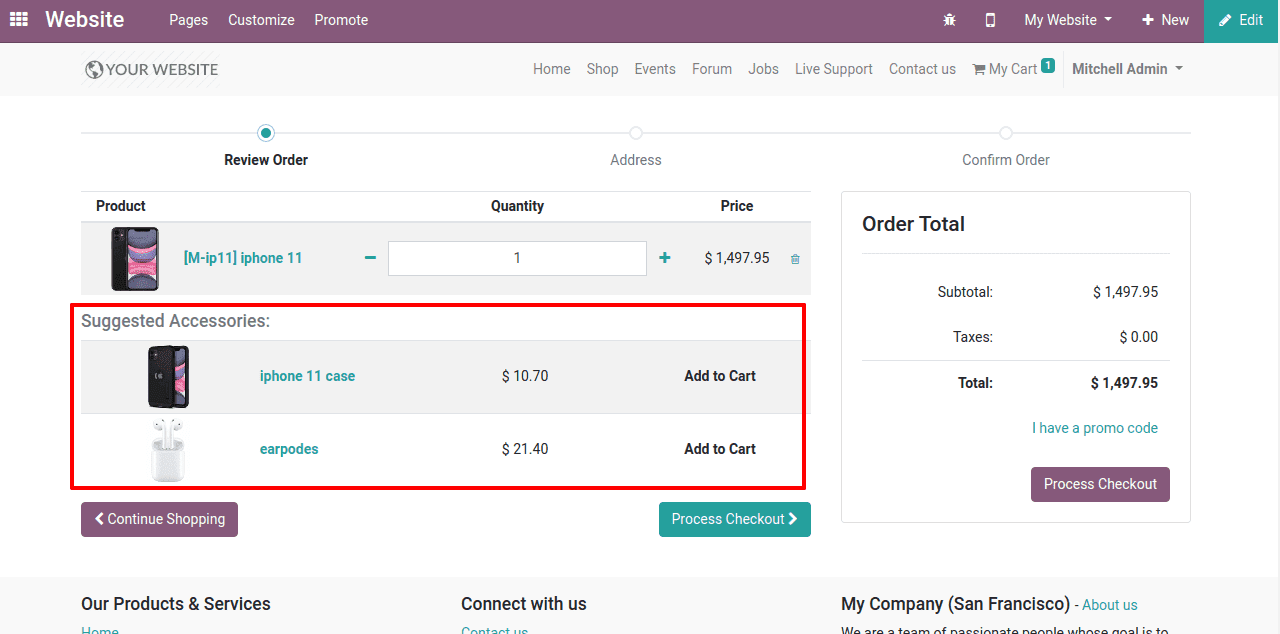This image is a screenshot from a website layout. The top half-inch of the image features a purplish header with a set of elements laid out systematically. In the top left corner, there's a 3x3 grid of smaller squares forming a larger square. The word "Website" is prominently displayed in bold white text, followed by smaller lettering that reads "Pages," "Customized," and "Promo."

On the top right corner, a greenish tab (with a teal hue) sits within the purple header, featuring an "Edit" text alongside a pencil icon. Adjacent to this, still within the purple header area, is a "New" label with a plus sign to its left, and icons for "My Website," "Cell Phone," and a bug-like icon.

Directly beneath "Website" on the left side, there is a globe icon accompanied by the text "Your Website." Below it, spaced about two inches down, lies a navigable list featuring sections like "Home," "Shop," "Events," and more, along with a total of six clickable options.

Further down, there's a green square followed by a white one that introduces "Mitchell & Men." Below this, a progress bar illustrates the user's ordering steps, starting about an inch in with "Review Order" indicated by a light green-filled circle. Centrally located on the bar is "Address," marked with an outlined circle, and to its right is "Confirm Order" with a partially filled circle.

Under this bar, columns titled "Product," "Quantity," and "Price" span across. Each product listed includes an image, description, quantity, and price details. Highlighting the product details is a prominent red rectangle.

Towards the bottom, the left side features a purple "Continue with Shopping" button, while a green-background "Process Checkout" button lies on the right. Under "Confirm Order," you'll find "Order Total," with sections for "Subtotal," "Taxes," and the final "Total." A promo code field is highlighted with a purple background and white letters, again with "Process Checkout" denoted at the bottom.